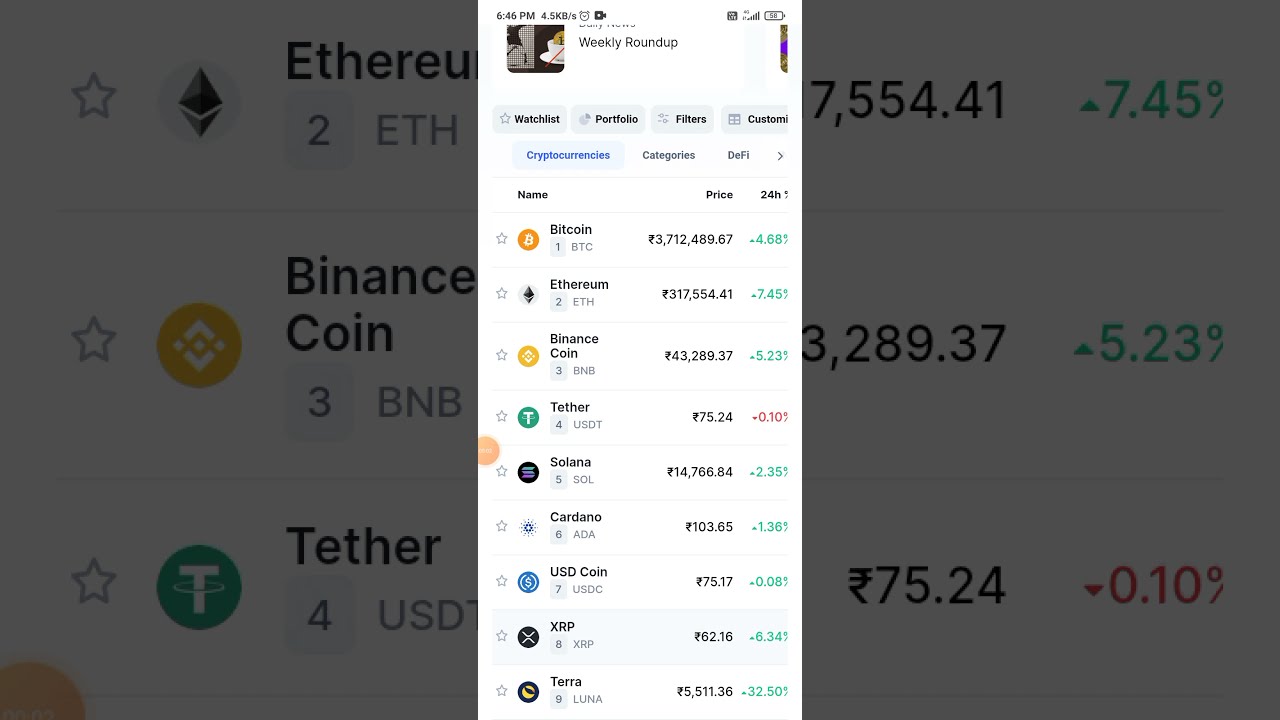This image is a very wide rectangular composition featuring a central, tall, rectangular screenshot from a cryptocurrency tracking app, flanked by darker close-up shots of the same screenshot on either side. At the top of the screenshot, there's a logo combining artwork and a cup with a yellow item in it, next to the black text "Weekly Roundup." Below this are several gray, rounded-rectangle buttons labeled with options. The main section of the screenshot displays an organized list of various cryptocurrencies, each presented with a star icon on the left, followed by the currency's logo, name, and symbol, alongside their current price. The listed cryptocurrencies include Bitcoin, Ethereum, Binance Coin, Tether, Solana, Cardano, USD Coin, XRP, and Terra. Additionally, the value change over the past 24 hours is indicated, with increases shown in green and decreases in red. The interface is designed to be clear and legible, suggesting it is a screenshot from an Android device, either a mobile website or an app for managing and tracking cryptocurrency investments.